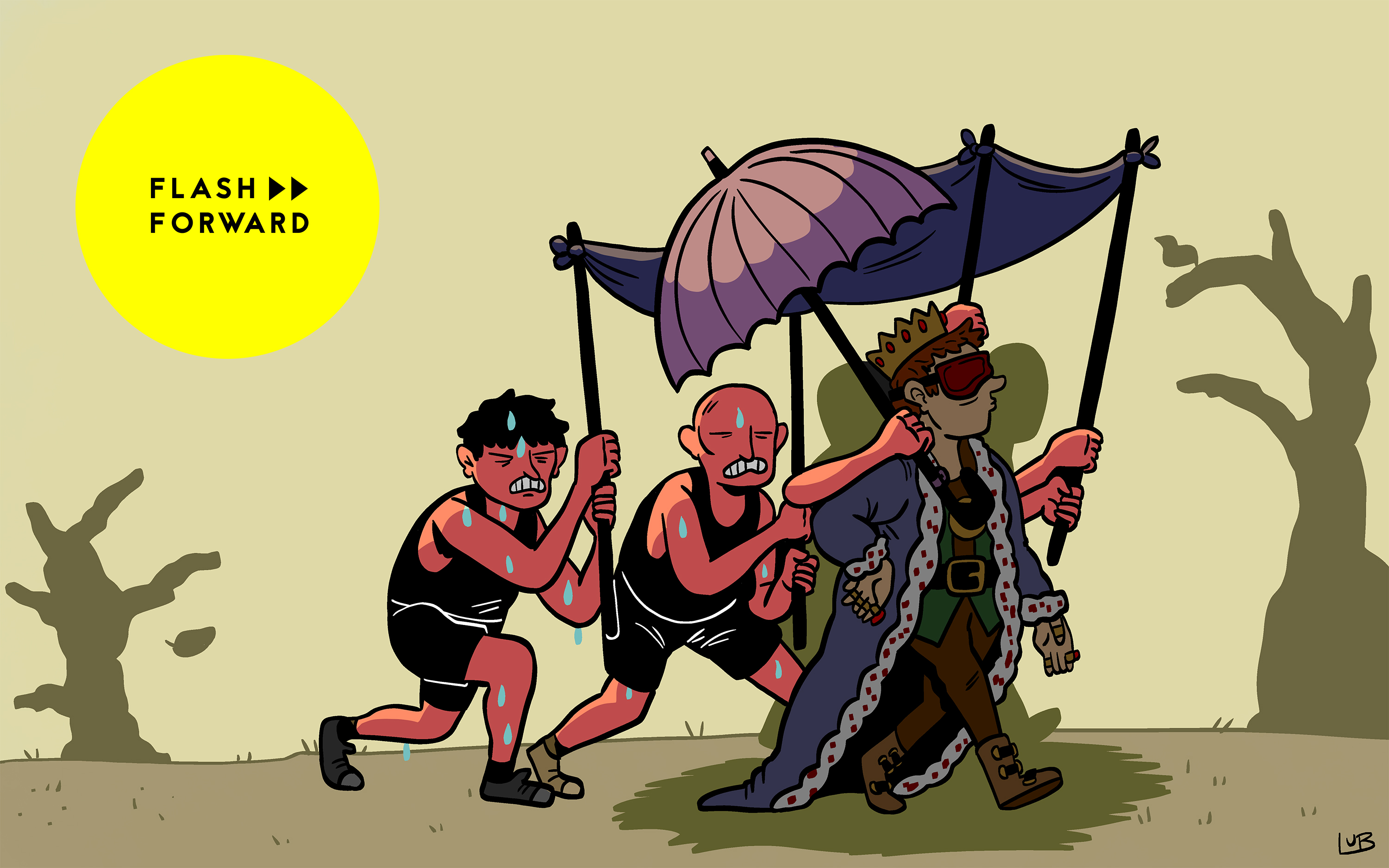In this colorful cartoon, presented from a landscape perspective, three men are walking towards the right side of the image. The first man, who appears to be a king, is elaborately dressed in a long purple robe trimmed with white fur. He dons a gold crown and visor-style sunglasses, adding an oddly modern touch to his royal attire. He is also wearing a green vest with a black belt, brown pants, and brown boots, resembling a leprechaun outfit. 

Behind the king, two muscular men are depicted in a beet-red hue, drenched in sweat, and wearing black and white singlets. These two men are visibly exerting themselves, with sweat dripping from their brows and pained expressions etched on their faces. They are carrying a large canopy over the king’s head to shield him from the scorching sun and are also holding an umbrella to ensure he remains entirely in the shade. 

Adding to the scene, a yellow circular banner with black text reading "Flash Forward" hovers in the background. The setting is a harsh desert, emphasizing the difficult conditions for the two men laboring behind the king while he remains comfortably shaded.